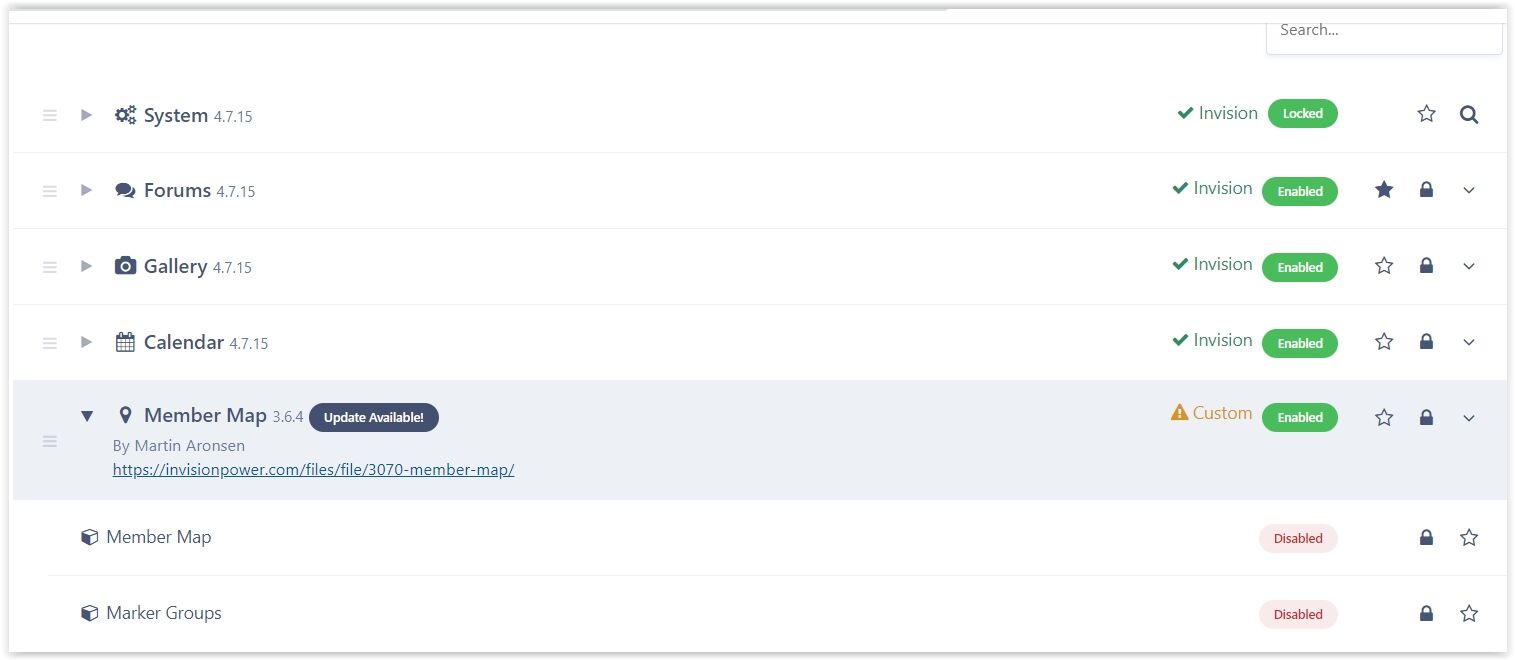Here is a cleaned-up and more detailed caption for the image:

---

A landscape-oriented screenshot of a website's interface showcasing various feature options in a wide layout. The interface has a column of options on the left side, each represented with icons, including hamburger menus and rightward-facing triangles. The fifth option down has been expanded, showing additional details as indicated by the downward-facing triangle.

The list, from top to bottom, includes:
1. System (version 4.715)
2. Forums (version 4.715) - this option is rated with stars.
3. Gallery (version 4.715)
4. Calendar (version 4.715)
5. Member Map (version 3.64 by Martin Aronson)

Each option, except the fifth, shows an adjacent "Envision" label with a green checkmark and green text denoting they are enabled. Notably, the Member Map option is marked with "Custom" in orange rather than "Envision". It also includes a blue URL link underneath the text, suggesting an update is available. The background of this section has a peach color.

Below this list, within the same section, are two additional options: Member Map and Member Groups, represented by cube icons and listed as disabled on the right side of the interface.

---

This caption provides a detailed and organized description of the image, enhancing its comprehensibility.